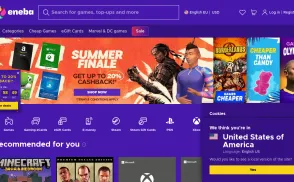This image is a screenshot taken from a website or app called Eneba, as indicated by the partially visible logo on the left side of a thick, medium-purple banner at the top. The banner also contains a search bar and several navigational icons, including options to choose a language, a heart button, a cart button, and an area for logging in or signing up.

Immediately below this, a thinner, darker purple banner with navigation options—written in small print and difficult to read—demarcates different sections of the site. The main content of the screenshot features a prominent image with the text "Save Big Under $5 Shop Now," accompanied by visuals likely representing various movies or games available for purchase. Directly below this promotional section, another segment titled "Recommended For You" is visible, along with a pop-up notification suggesting the user is located in the United States of America. The overall page is set against a purple background, and the screenshot's small size makes some details challenging to discern.